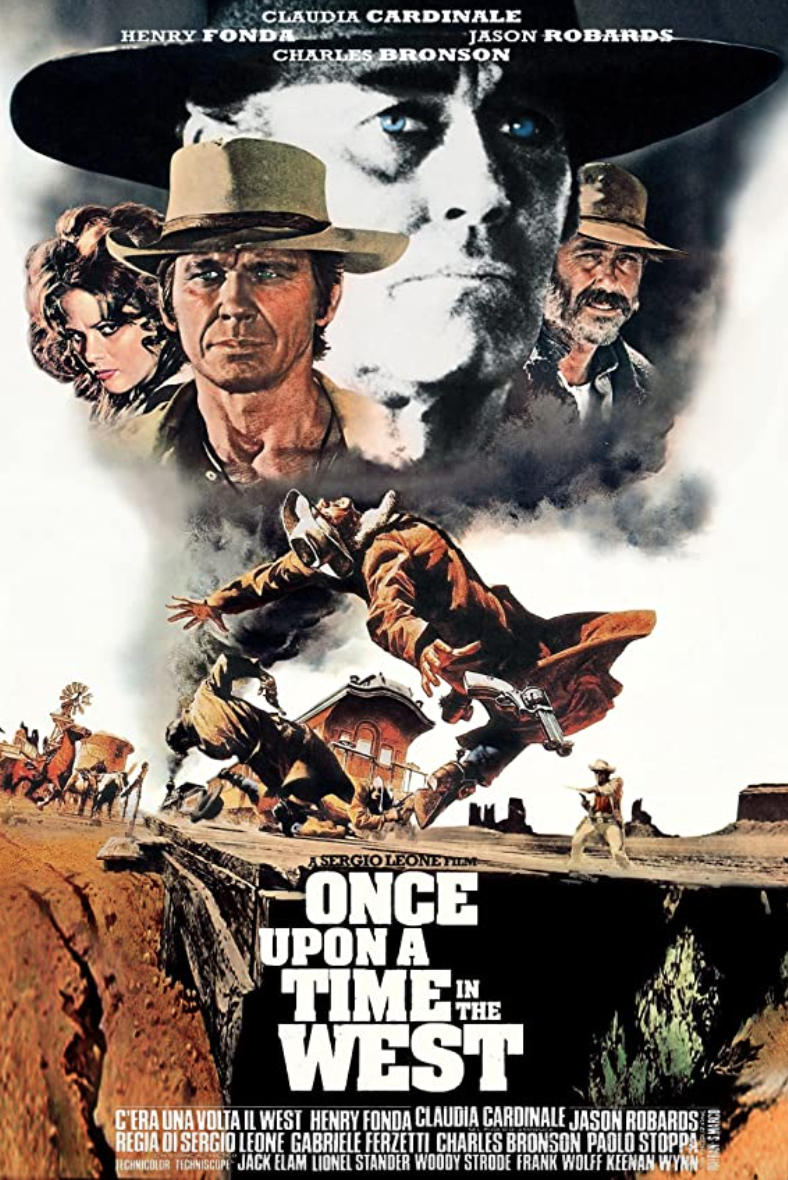This is a highly detailed movie poster for Sergio Leone's classic western film, *Once Upon a Time in the West*. At the top of the poster, prominent white text lists the main actors: Claudia Cardinale, Henry Fonda, Jason Robards, and Charles Bronson. Below their names are their images, with Charles Bronson's picture considerably larger and in black and white, while the others are in color. The headshots appear to emanate from the top of a plume of smoke or tornado, which spirals downward toward a scene dominated by a train.

In the middle section of the poster, a dramatic gunfight unfolds with cowboys dueling near train tracks, guns blazing, and horses charging in the dust-filled air characteristic of a wild west setting, likely Arizona or New Mexico. This vividly illustrates the intense action typical of Leone's western epics.

Near the bottom, in bold white font, is the film's title, *Once Upon a Time in the West*, further emphasized by smaller white text listing the actors’ credits. The poster, rendered in a hyper-realistic hand-drawn style, exudes a vintage 1970s feel, capturing the gritty essence of the western genre.